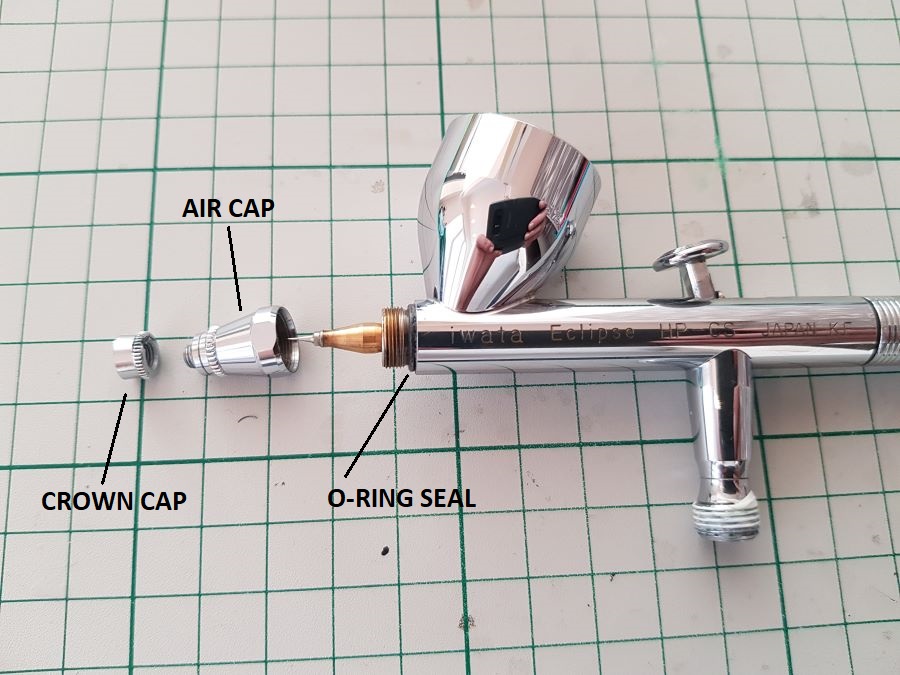The image is a detailed photograph of an airbrush tool, set against a green graph paper background. The chrome airbrush, reflective enough to glimpse the photographer’s hands holding a phone, is organized with some of its parts labeled. Prominent labels in black text include the "crown cap," a knob-like component at the left end; the "air cap," a funnel-shaped piece adjacent to it; and the "O-ring seal," a thin blue washer near the base of the airbrush.

The main body of the airbrush, which holds the pinpoint nozzle with a light brown base and a screw top where the air cap is attached, is visibly prominent but not fully labeled. A small cup, likely for paint, is welded onto the top near the nozzle. The airbrush features intricate details like a chrome button used to control airflow and a threaded extension at the base for attaching an air tube. The airbrush is etched with markings indicating it is an "Iwaha Eclipse HP-G6" model and made in Japan, with "Japan KC" clearly visible on the right side. The meticulous arrangement of parts on the graph paper suggests it could be a page from an instruction booklet, highlighting only key components while leaving other visible parts unlabeled.